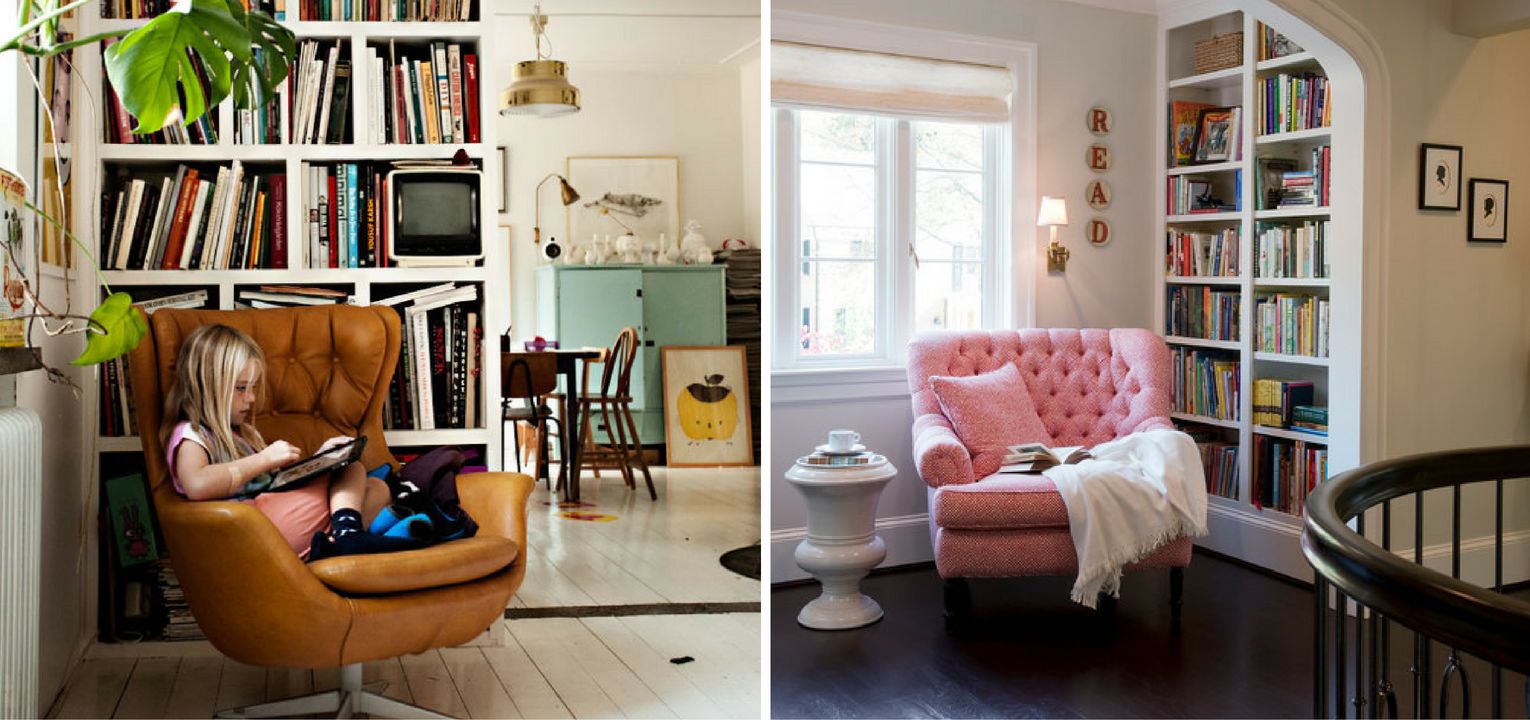The composite image displays two side-by-side photos, each capturing distinct, yet similar, indoor settings. 

In the left photo, a young blonde girl is seated on a brown leather lounge chair with a white base in the corner of a room. She is dressed in pink and has a blue and black throw beside her, absorbed in a tablet. Behind her is a white bookshelf filled with various books and a small TV on one of its shelves. The background reveals white walls and white hardwood flooring extending into a distance where a dining table with a golden chandelier and a blue dresser are partially visible. A plant is positioned by a window on the left side of this photo, adding a touch of greenery.

The right photo features a pink lounge chair situated catty-corner in a room, placed in front of a window. A white table stands next to the chair, and there's a white bookshelf behind it housing an array of books. The decor includes a series of mounted circles on the white walls, spelling out "R.E.A.D." in red letters. The floor is made of dark mahogany hardwood, contrasting the lighter tone of the other room. A stairwell with a dark railing is visible on the right side, accompanied by two framed photos leading down a hallway. The setup reflects a space likely on the second floor of a house, with abundant natural light streaming through the window.